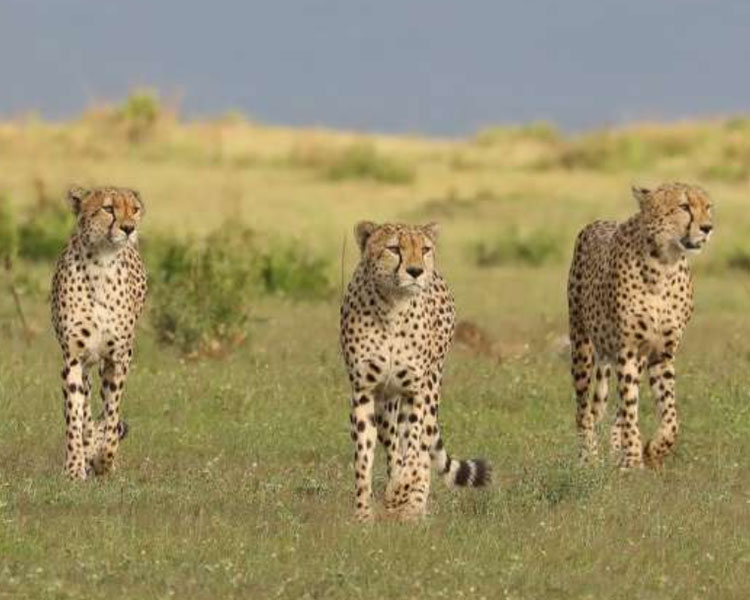This captivating photograph showcases three cheetahs, likely siblings, standing together on the African savannah. The cheetahs are positioned with one on the left, one in the center, and one on the right, all facing slightly to the left, fixated on something outside the frame. Their bodies are turned towards the viewer, offering a clear view of their sleek, spotted coats characterized by a yellowish-brown hue and distinctive black markings. The central cheetah's tail extends out to the right, displaying a pattern of white with black stripes. The cheetah on the far right has its mouth slightly open, adding to the impression they are hunting. They stand on a bed of green grass, punctuated by rough, small shrubbery, with a blurred background that suggests a gentle rise, indicating they are amidst the rolling hills of the savannah. The setting, captured in a medium gray light, emphasizes their lush environment and the tense focus of these majestic predators, likely in the midst of tracking their next meal.